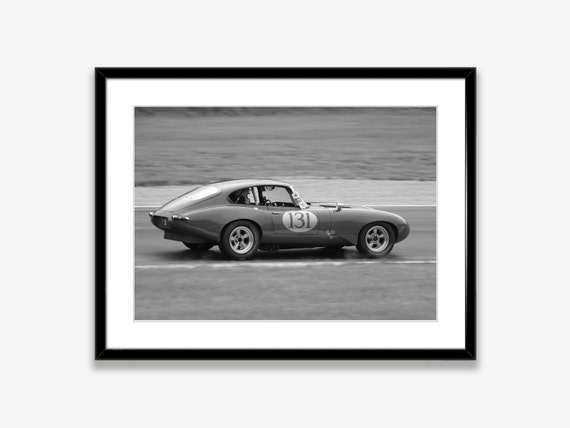Framed elegantly with a thin black rim and a one-inch white border, this black and white photograph captures an old race car in motion. The vintage vehicle, marked with the number 131 within a white oval on its door, exudes a classic charm. Its design, reminiscent of a Corvette with a Porsche-like rear, suggests it might be an import car. Positioned on what seems to be a track, the background appears slightly blurred, hinting at the car's speed, with indistinct surroundings that could be either fields or water. A faint silhouette of the driver is visible inside the car. The frame hangs on an off-white, grayish wall, adding to the picture's nostalgic allure.